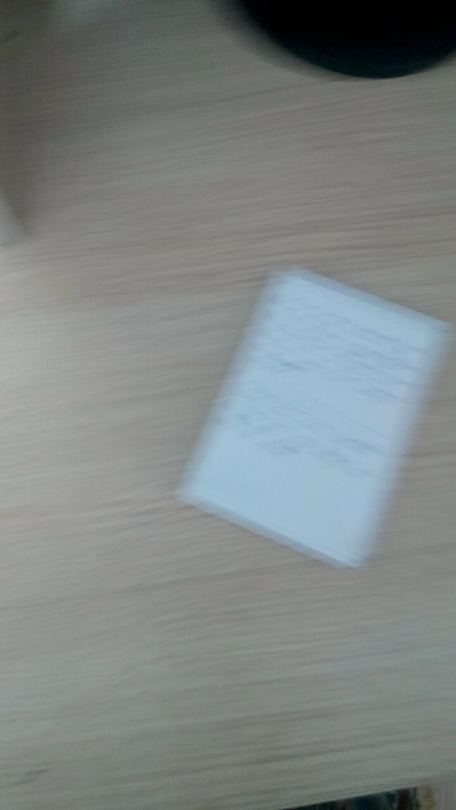In this blurry photograph, the scene appears to be set upon a desk or table. The central focus is on a piece of paper, featuring handwritten text arranged into two discernible paragraphs, though the content remains indecipherable due to the image's lack of clarity. Surrounding the paper are various indistinct objects, among which a black, rounded item stands out, though its exact nature remains unclear. Additionally, a laptop with some items atop it can be faintly seen, further adding to the cluttered yet intriguing tableau of an active workspace.